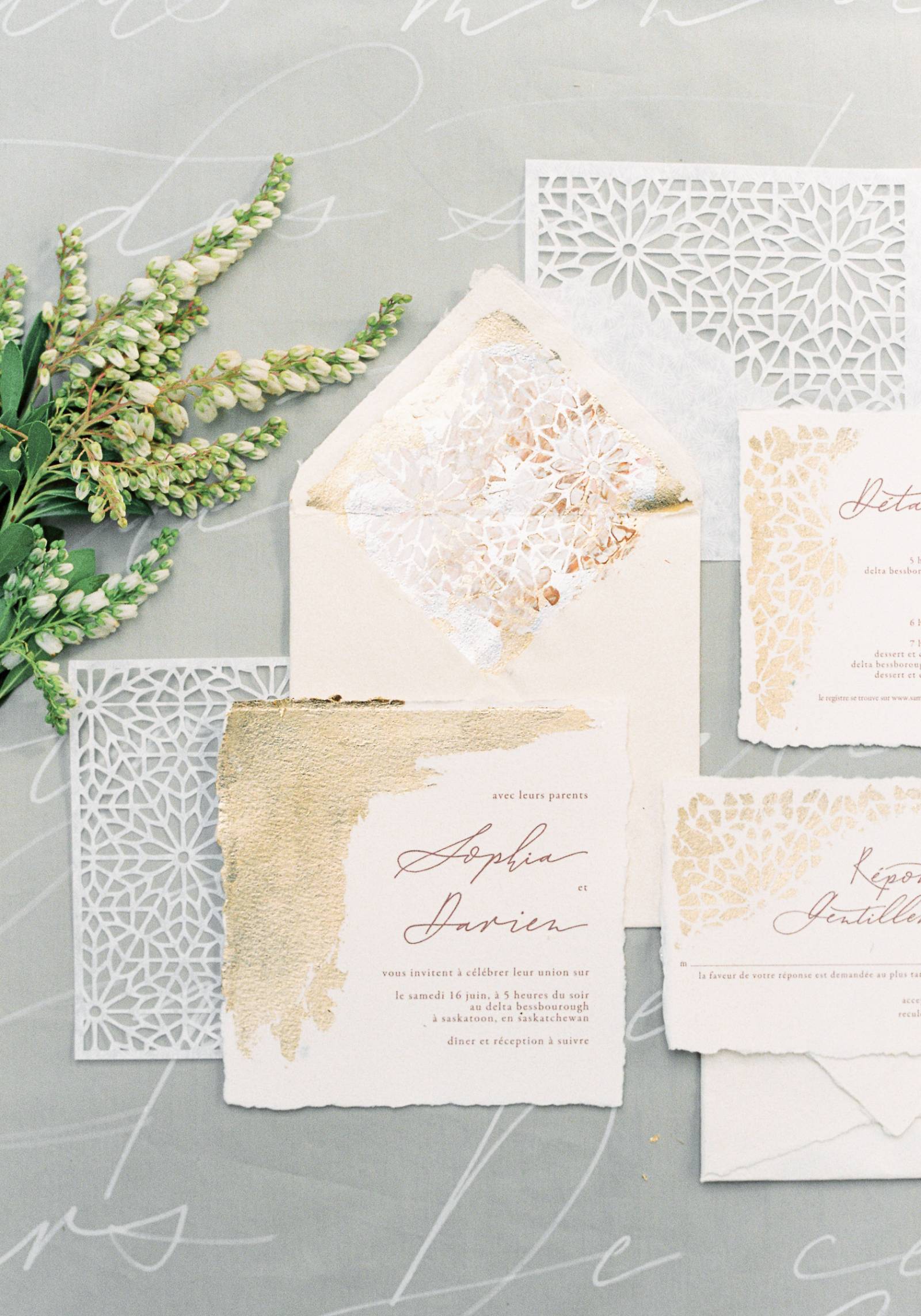This photographic image showcases an elegantly styled invitation set, featuring an envelope and several note cards adorned with sophisticated text. The central note card prominently displays the names "Sophia and Darren" in a mix of English and French, adding a touch of international flair. The envelope, in muted milk and brown tones, sits above and behind the note card, creating a layered effect. Nearby, additional note cards are positioned to the right and top right of the main focus. A delicate white paper pattern with an intricate flower design enhances the top right corner, while a cluster of unbudded green flowers adds a natural touch to the scene. The background, a gray surface with subtle white lined markings, provides a refined backdrop that complements the color scheme of white, brown, green, and hints of red. The overall composition is thoughtfully arranged to highlight the sophisticated design of the invitation suite.